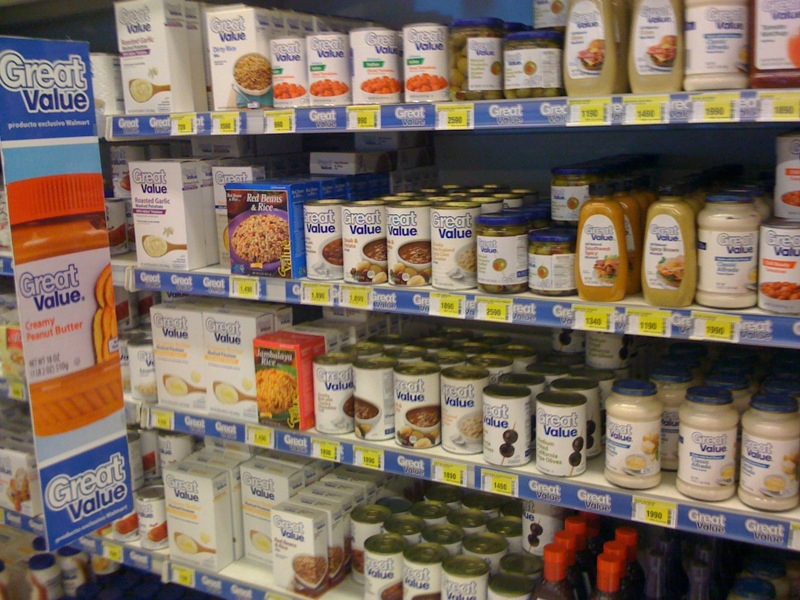The image depicts an aisle in a Walmart supermarket, identifiable by the prominent Great Value brand on various products. The shelves are stocked with a diverse array of food items, including canned goods, condiments, and packaged foods. Visible products include canned chili, red beans and rice, diced carrots, and jars of green and black olives. Numerous plastic bottles of ketchup, jars of pasta sauce, honey mustard, and mayonnaise are also present. On one side, there is a notable vertical banner with a blue-bordered sign displaying a container of creamy peanut butter under the Great Value brand. Multiple yellow price tags can be seen along the shelves, further emphasizing the commercial setting.